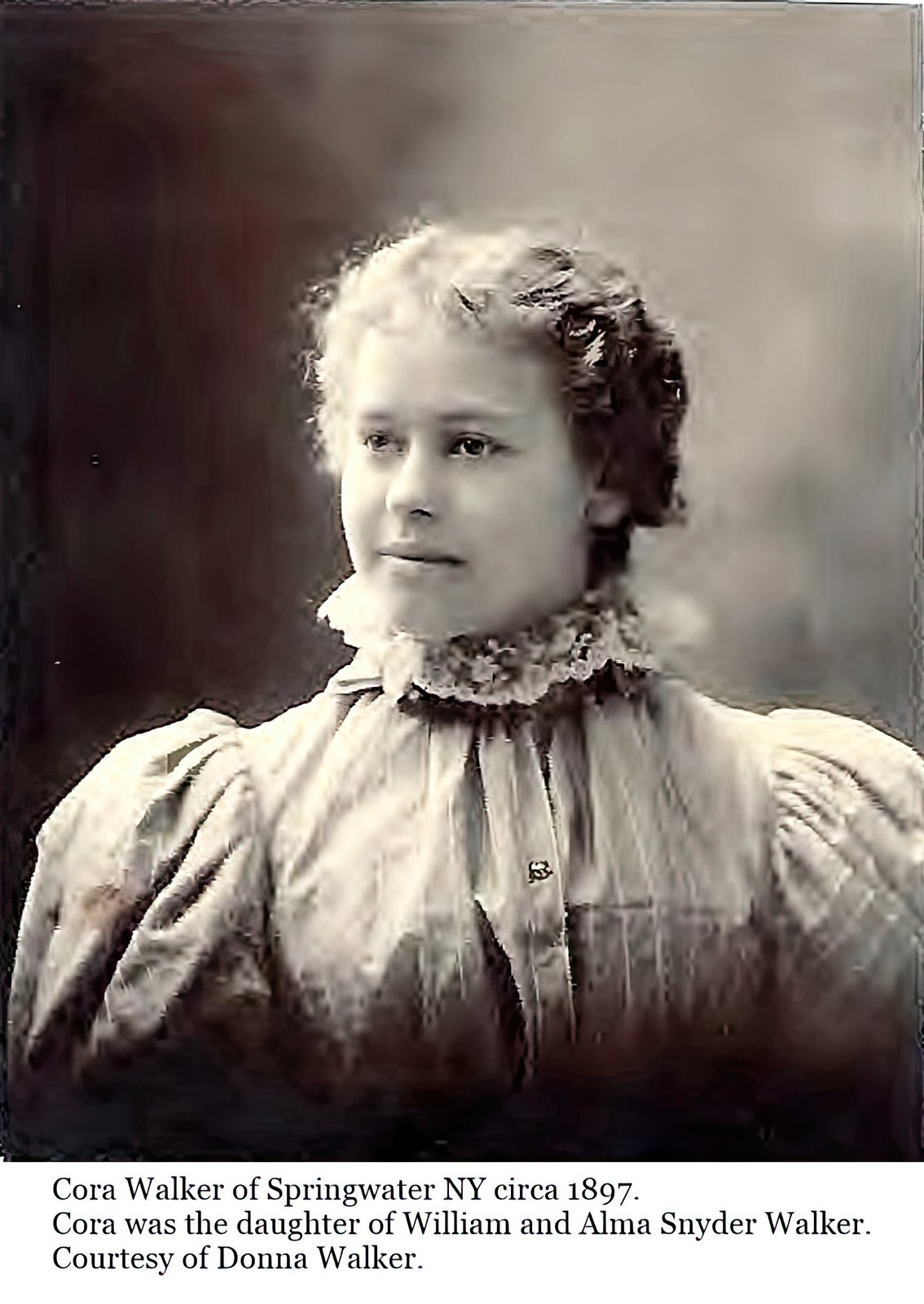This black-and-white photograph from 1897 features a young woman named Cora Walker from Springwater, New York. Cora, the daughter of William and Alma Snyder Walker, is poised in a dress reflective of the late 19th century fashion, characterized by its puff sleeves and a high lace collar that reaches up to her chin, adorned with floral frills. Her hair is neatly pulled back into a bun, accentuating her youthful face. The photograph captures her gazing off to the left, with a stream of sunlight illuminating one half of her face, giving her an ethereal, almost angelic appearance. The background is simple, darker on the left side, contrasting with the bright light that highlights her features. The image exudes a timeless beauty, enhanced by the historical context provided by Donna Walker.